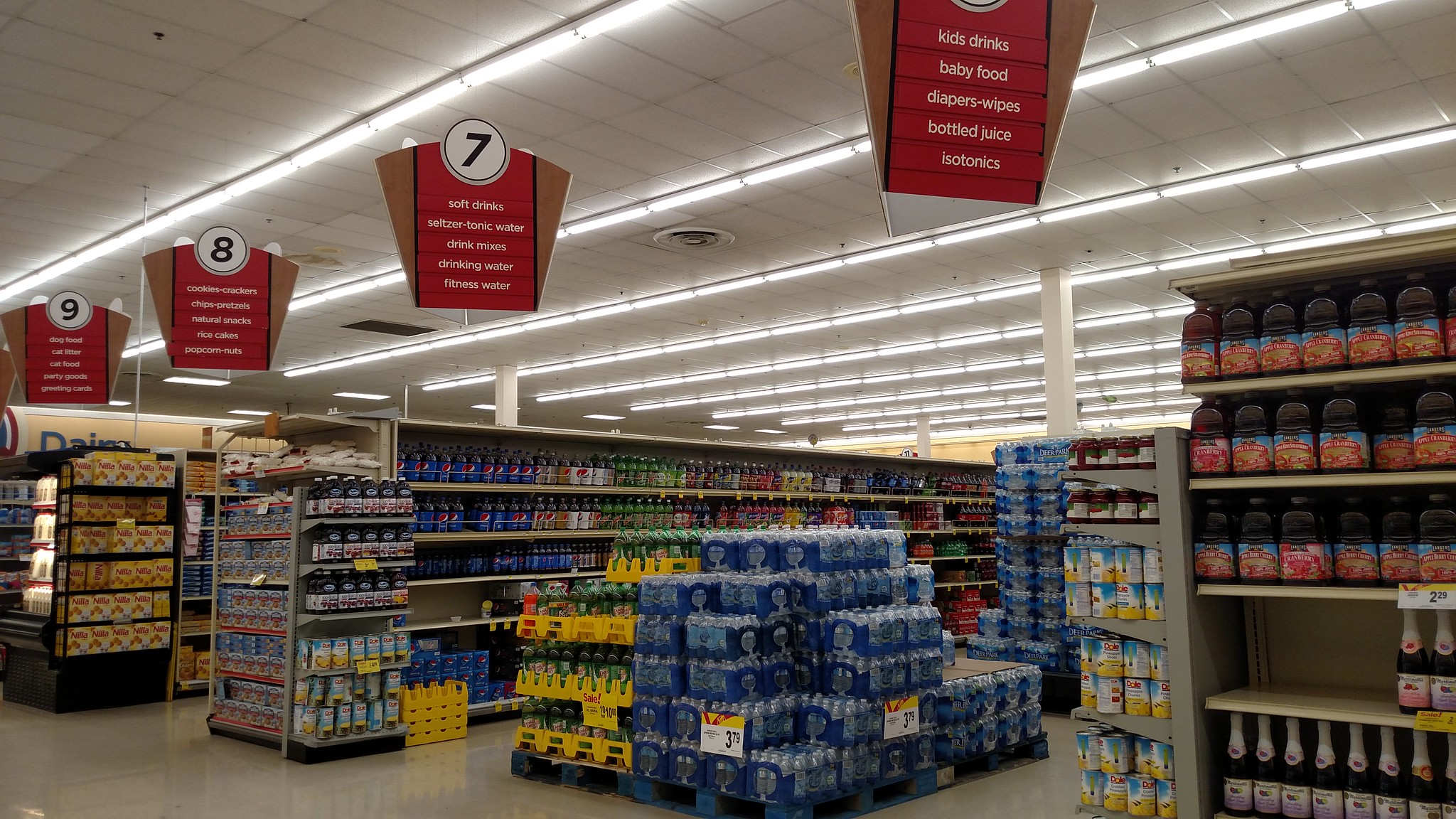This detailed photograph captures the interior of a well-lit grocery store, focusing on various aisles stocked with a diverse array of items. The image prominently features aisle number six, which is marked by a red sign with white font, listing items such as kids drinks, baby food, diapers and wipes, bottled juice, and isotonics. Adjacent to it is aisle number seven, indicated by a similar sign that lists soft drinks, chips, drinking water, wine, and more.

In the center of the aisle, there is a noticeable stack of water bottle cases in white, dark blue, and light blue packaging. These cases are wrapped in plastic and have a $3.79 sticker on them. Next to the water bottles, there are green beverage bottles organized in yellow holders. The shelves to the right display various beverages, including the soda brands Pepsi and Mountain Dew, along with sparkling and regular juice.

On a side shelf, Dole canned fruit is also visible. Above, the ceiling is lined with overhead fluorescent lighting that provides ample illumination throughout the store. This bright lighting helps highlight the well-stocked shelves and the organized flow of the aisles, creating a clean and inviting shopping environment.